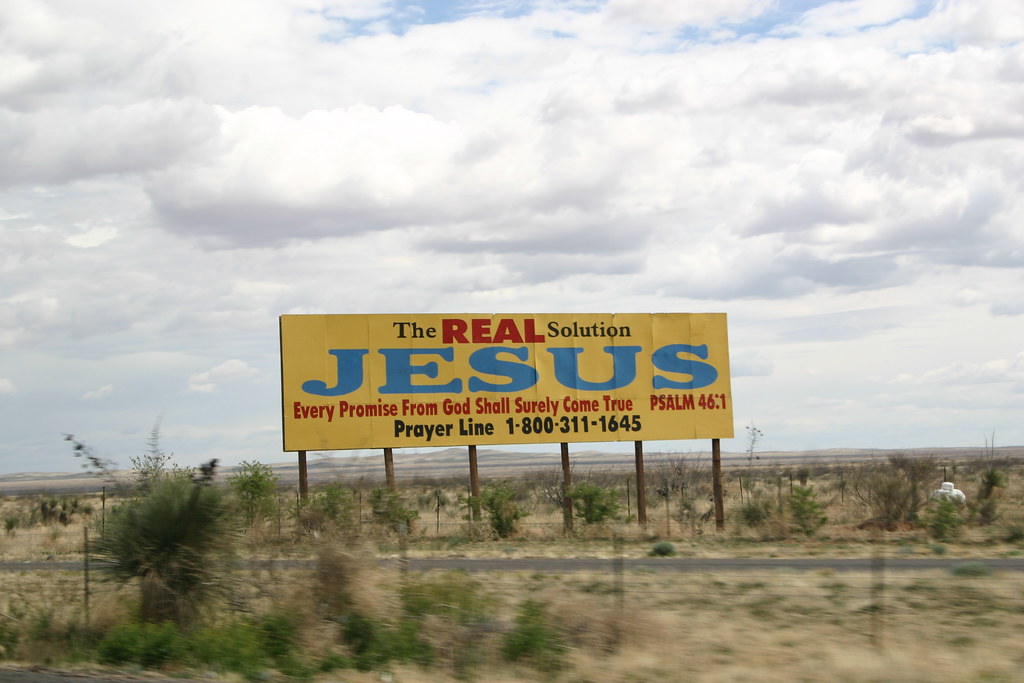In this color photograph taken outdoors, a large rectangular yellow billboard stands prominently against a desolate, desert-like setting. The billboard, supported by six wooden posts, features the text "The real solution" with the word "real" in bold red letters, followed by "Jesus" in large, wide blue letters. Further down, it says, "Every promise from God shall surely come true" in red text, accompanied by the citation "Psalm 46:1" and a prayer line number "1-800-311-1645" in black lettering. The setting is barren with mostly brown ground and scattered small green shrubs, likely weeds or dead grass. In the far background, desert mountains rise under a blue sky filled with numerous puffy white and gray clouds. A narrow, gray roadway runs horizontally near the base of the billboard. The sky occupies the upper three-quarters of the image, adding to the expansive and remote atmosphere of the scene.